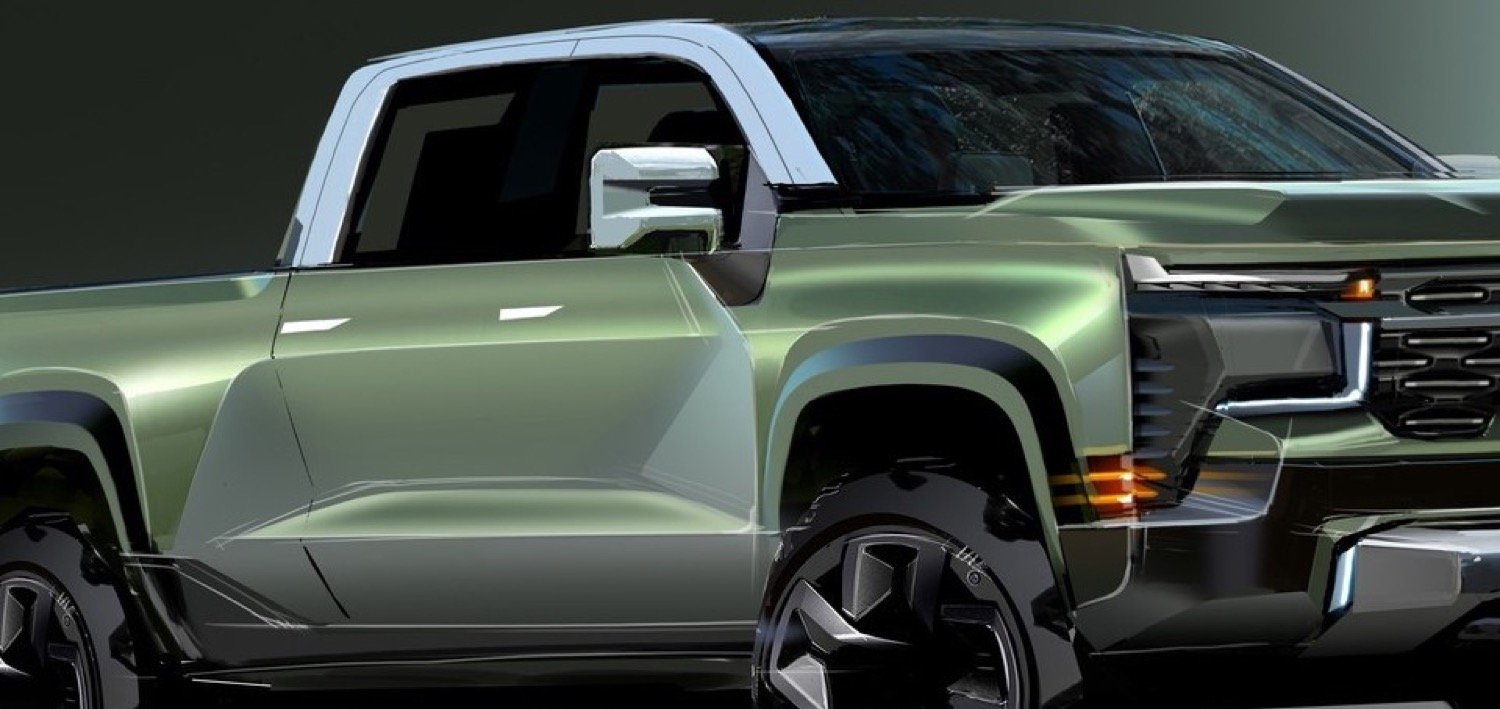The image depicts a high-tech, possibly AI-generated or graphically designed, concept art of an olive green pickup truck with single or possibly double cab. The truck is shown at an angle, revealing the front right corner and the left side. The passenger door and side view mirror feature gray-blue trim, while the dark background gradients from black to a lighter gray on the right, suggesting a light source from that direction. The truck's windshield is sharply slanted, and the door has rectangular indentations with triangular shadows creating shelf-like illusions. The bottom half of the right-side wheels is visible, adorned with angular hubcaps and black tires. Yellow sub-headlights are situated beneath the main, darkened headlight on the right, encased in white trim. The front grille and bumper are also prominent, adding to the stylish, rugged appearance of this green-hued vehicle.